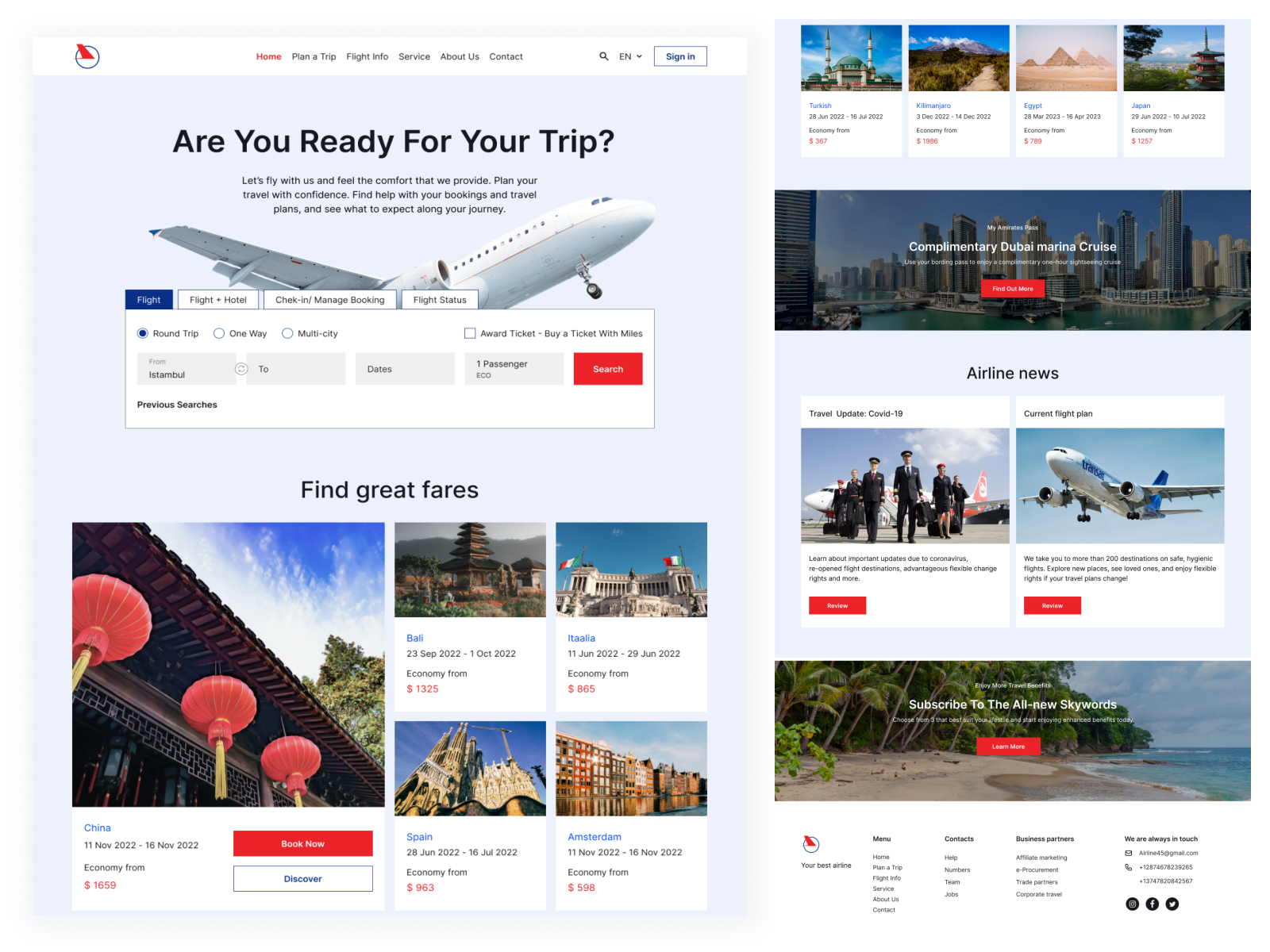This image, sourced from a website, showcases a bird-like icon encircled in red, reminiscent of an airplane logo, against a faint light blue background. Above the logo is a sleek navigation bar with the following menu items listed sequentially in red ink: "Home," "Plan a Trip," "Flight Info," "Service," "About Us," and "Contact." To the far right of the navigation bar, a magnifying glass icon is followed by the text "EN" with a dropdown menu for language selection, next to a blueprint-colored "Sign In" button.

Dominating the center of the image is a large, impressive airplane accompanied by an inviting message: "Are you ready for your trip? Let's fly with us and feel the comfort that we provide. Plan your travel with confidence. Find help with your bookings and travel. Make plans and see what to expect along your journey."

Beneath this, a comprehensive interactive section allows users to select options for booking flights and hotels, check flight status, find great fares, and stay updated with airline news. The image is enriched with various pictures, enhancing the user experience, and concludes with a subscription invitation to the airline's newsletter, "Sky Words."